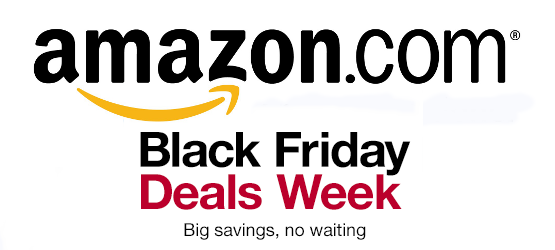This image is a screenshot from Amazon.com, showcasing a promotional banner on a completely black background. At the top, "amazon.com" is prominently displayed in large, bold black text. To the right of this text is an "R" enclosed in a circle, indicating a registered trademark. Beneath "amazon.com," the yellow Amazon smile logo is visible, adding a touch of color to the image.

Below the logo, three lines of text further emphasize the promotional message. The first line reads "Black Friday" in bold black text, capturing immediate attention. The second line states "Deals Week" in vibrant hot pink, highlighting the duration of the event. The third line, in smaller black text, assures potential customers of "big savings, no waiting," all set against a solid white background for stark contrast.

The absence of scroll bars, side elements, or additional images keeps the viewer's focus purely on the details of the promotional offer. This clean, straightforward layout effectively communicates the exciting Black Friday deals available on Amazon.